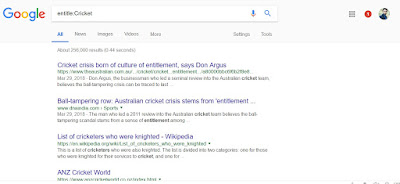This is a detailed caption for the described image:

"A desktop screenshot of a Google search results page. The search query includes the word 'cricket', although the first word is hard to discern. The search results focus on cricket stories and articles related to Australian cricket, with the final entry mentioning 'ANZ cricket world' and 'Australia' in the link. The screenshot shows a user logged into their Google account, evidenced by a small, low-resolution circular profile picture and an initial in the top right corner. The Google logo is clearly visible in the top left. The interface is straightforward, with the search bar at the top and text-based search results centered below it."